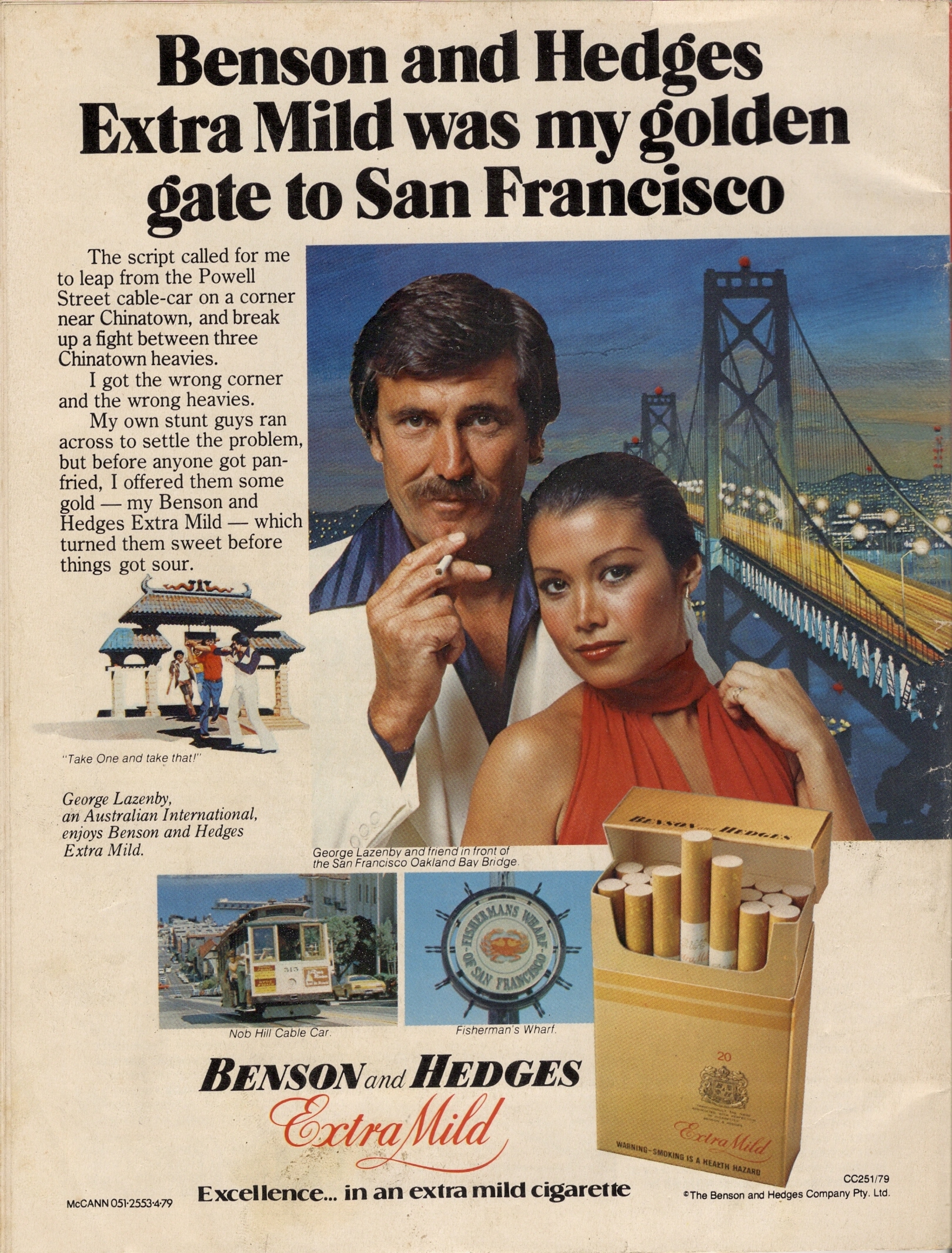The image is an old 1970s magazine advertisement for Benson and Hedges Extra Mild cigarettes. It features a white middle-aged man with thick mustache and brown, slightly graying hair, dressed in a white polyester suit reminiscent of the "Saturday Night Fever" style, complete with a large blue butterfly lapel and an open collar revealing a bit of chest hair. He holds a cigarette in his right hand, pinched between his middle and index fingers, not quite to his mouth. Next to him stands a younger woman with black hair, possibly of Italian, Native American, or other White descent, identified by her tanned skin with a brownish hue. She wears vibrant makeup and red lipstick, donning a striking red-orange dress that wraps around her neck and falls across her chest like a scarf. She has a ring on her pinky finger.

Behind them is a painting of a San Francisco bridge, likely not the Golden Gate but one of the others in the area, establishing the setting. The advertisement prominently features a gold carton of Benson and Hedges Extra Mild cigarettes with a few cigarettes propped up in the middle. A crest adorns the bottom right of the carton, with "Extra Mild" written in red cursive beneath it.

Text at the top in bold black lettering announces, "Benson and Hedges Extra Mild was my golden gate to San Francisco." Below in script, a narrative unfolds: "The script called for me to leap from the Powell Street cable car on a corner near Chinatown and break up a fight between three Chinatown heavies. I got the wrong corner and the wrong heavies. My own stunt guys ran across to settle the problem, but before anyone got pan-fried, I offered them some gold—my Benson and Hedges Extra Mild, which turned them sweet before things got sour."

A small image depicts a man in a similar outfit as the main character, involved in a dramatic scene with two other men, possibly related to the narrative, next to a structure resembling a Chinese temple. Underneath, it reads, "Take one and take that," with an additional note identifying the man as George Lazenby, an Australian international, enjoying Benson and Hedges Extra Mild.

Two small photographs also feature iconic San Francisco landmarks, a cable car, and Fisherman's Wharf logo, further grounding the scene in San Francisco's cultural landscape. Beneath these images, the text reads "Benson and Hedges Extra Mild" in varying fonts and sizes, with "Excellence... in an extra mild cigarette" at the very bottom, accompanied by small text detailing the company's information on the lower edges.